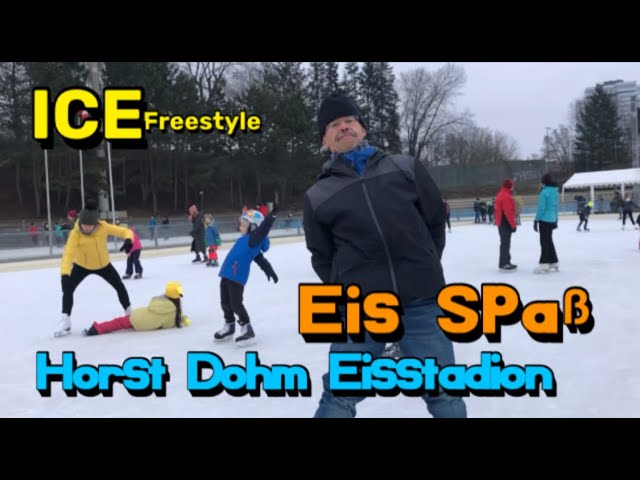This color photograph captures a lively and bustling scene at an outdoor skating rink. In the foreground, a man wearing a black jacket, black knit cap, and jeans stands slightly leaning to his right, looking directly at the camera with a mustache and glasses, giving a faint smile. Surrounding him, numerous adults and children in varied attire—parkas, snow pants, and coats—are enjoying their time on the ice. To the left of the man, there is a girl in red pants who has fallen, and a man is helping her up. In the background, people can be seen skating and chatting amidst the wintery backdrop of trees and a whitish sky. Towards the right, there is a building and a snowshed. The photograph features text in black bands at the top and bottom. The upper left corner reads “Ice Freestyle” in yellow text, while at the bottom, “Horst Dorf Eistadion” and the word “E-I-S-S-P-A-B” in blue text indicate information in another language, possibly Nordic.